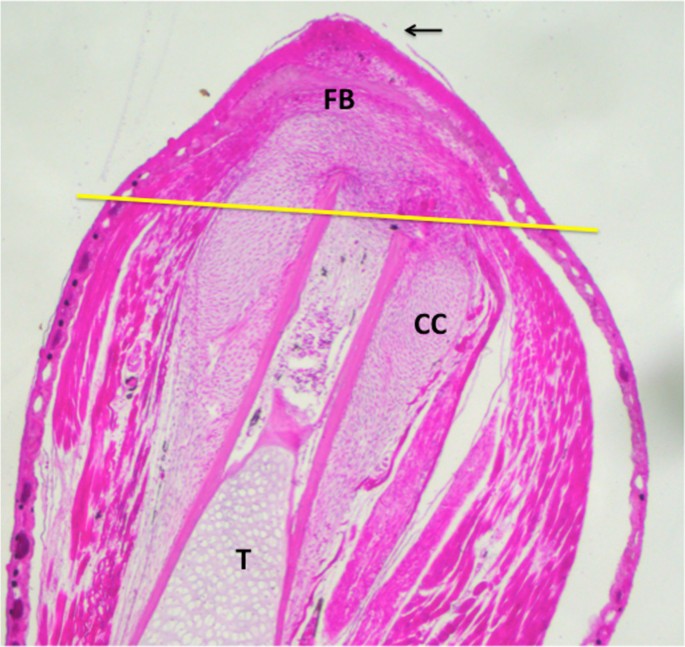This detailed microscopic image reveals a complex structure, possibly some form of tissue. The object, which has a shape reminiscent of a halved lemon or football, features a pinkish-purple or fuchsia hue and is covered with numerous fine lines and streaks, contributing to its intricate appearance. At the very top of the structure, where it comes to a slight point, a black arrow points from right to left towards a small protrusion labeled "FB" in black letters. Additionally, the image contains labels such as "CC" on the right side and "T" below it, indicating different areas within the sample. A thin yellow horizontal line, positioned about a third of the way down, seems to divide the upper and lower sections of the specimen. Overall, the image is densely packed with details and labeled sections, making it informative yet challenging to identify without expert knowledge.